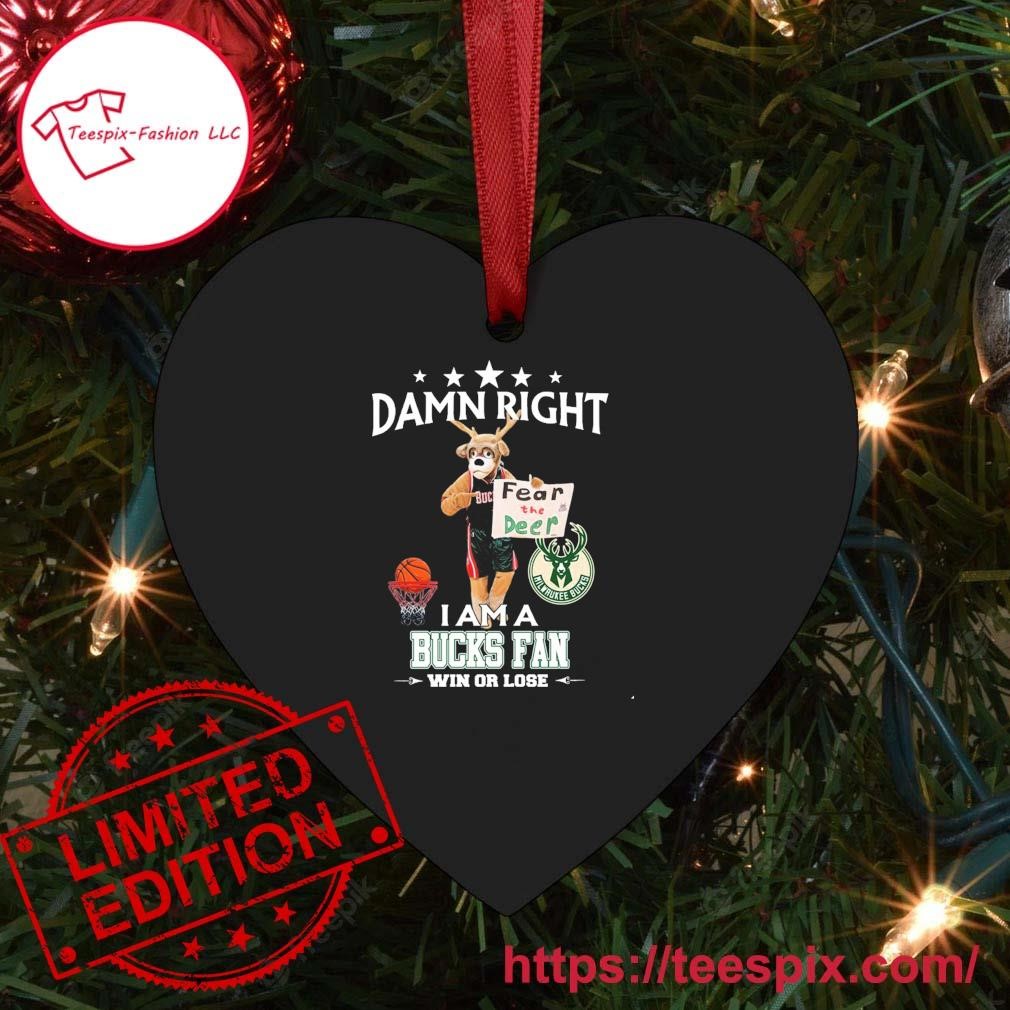The image showcases a close-up of a heart-shaped black Christmas ornament hanging on an artificial, pre-lit Christmas tree. The ornament prominently displays the text, "Damn Right I'm a Bucks fan win or lose," with an image of the Bucks mascot, a deer dressed as a basketball player, holding a sign that reads "Fear the Deer." The background highlights the tree branches adorned with small lights, enhancing the festive atmosphere. In the top left corner, a white circle outlined in red contains the text "Tees Picks - Fashion LLC" along with a cartoon outline of a shirt. Additionally, a bold, red "Limited Edition" stamp with stars above and below is situated at the bottom left of the image, and the website "teespix.com" is also visible, indicating where this exclusive ornament can be ordered.